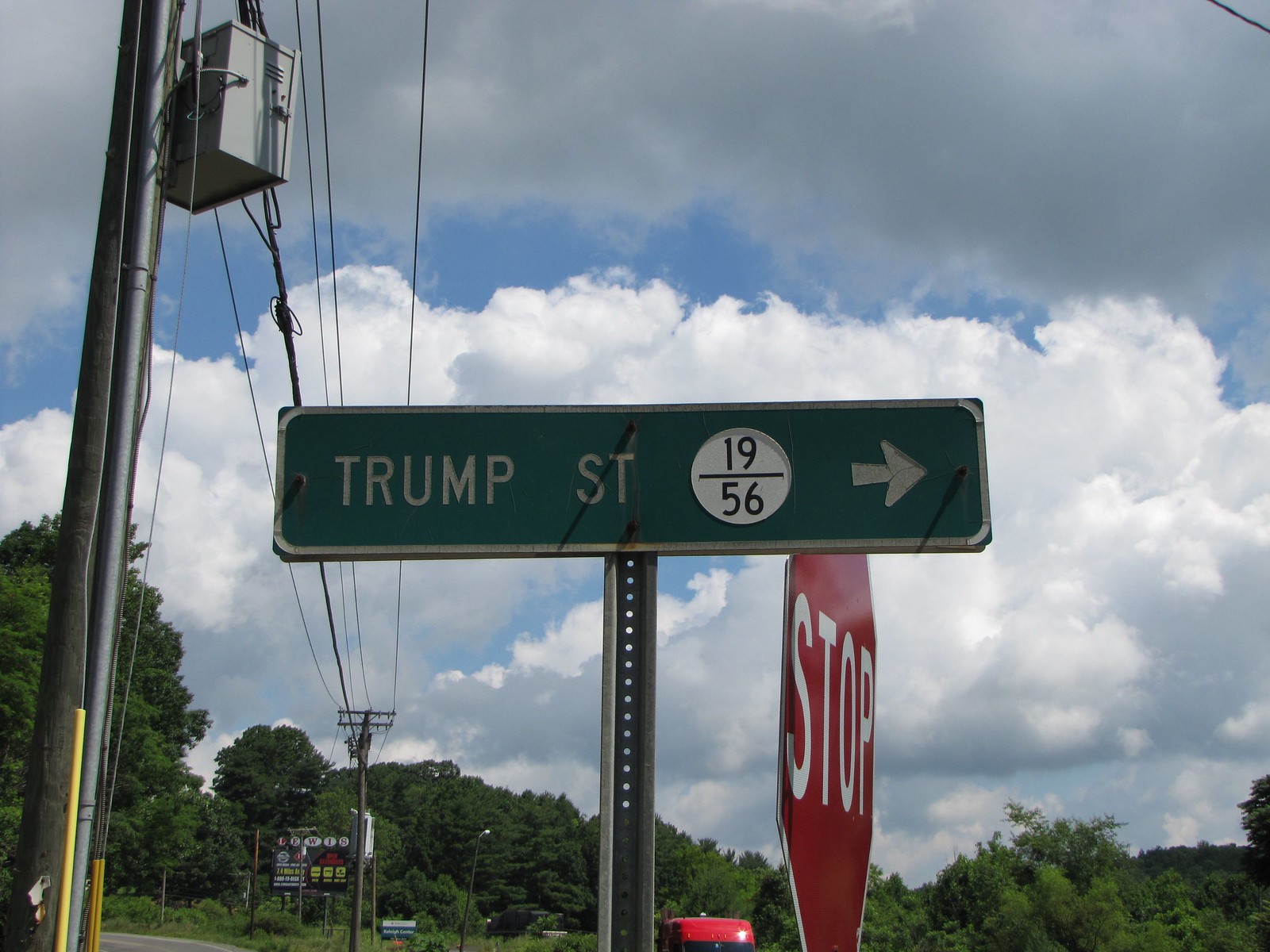A rectangular image with a landscape orientation features a street scene as its main focus. Dominating the center of the image is a rectangular street sign, mounted on a metallic pole punctuated with evenly spaced holes. The street sign has a green background with a white border and white text, reading "Trump Street 19 over 56" accompanied by an arrow pointing to the right. To the bottom right of this street sign, a slightly angled stop sign displays its white "STOP" text on a red background, although not directly facing the viewer. On the left side of the scene stands a tall wooden telephone pole, extending vertically from the bottom to the top of the image, with what appears to be a transformer affixed near its upper section. Enhancing the composition, the background showcases a predominantly cloudy blue sky with a vibrant stretch of green trees occupying the lower portion of the frame.